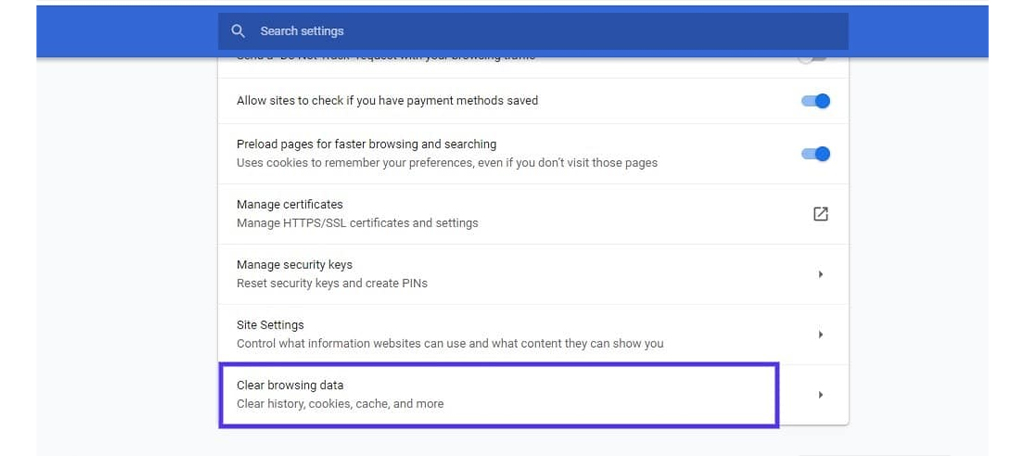The image appears to be a screenshot from a Google product, likely the settings menu of the Google Chrome web browser on a computer. The interface is expansive, indicating it covers the width of a desktop screen. The primary focus is on the "Search settings" section, although the upper part of the screen is not fully visible.

Within this visible portion, several options are listed, each enabling users to control different aspects of their browsing experience. Specifically, the settings shown are:

1. **Allow sites to check if you have payment methods saved:** The option is enabled (indicated by "Yes").
2. **Preload pages for faster browsing and searching:** This is also enabled (indicated by "Yes").
3. **Manage certificates:** Offering users the ability to handle their digital certificates.
4. **Manage security keys:** Allowing control over security keys used for two-factor authentication.
5. Other settings, possibly related to site permissions, although the text is partially obscured and therefore hard to read.

At the bottom, there is an option to **control what information websites can use and what content they can show you**, indicating the section is likely about site settings.

Finally, the option to **clear browsing data** is prominently highlighted by a blue bar, suggesting the possibility to remove history, cookies, and cached data.

These features collectively provide users with extensive control over their privacy and security settings within the browser.